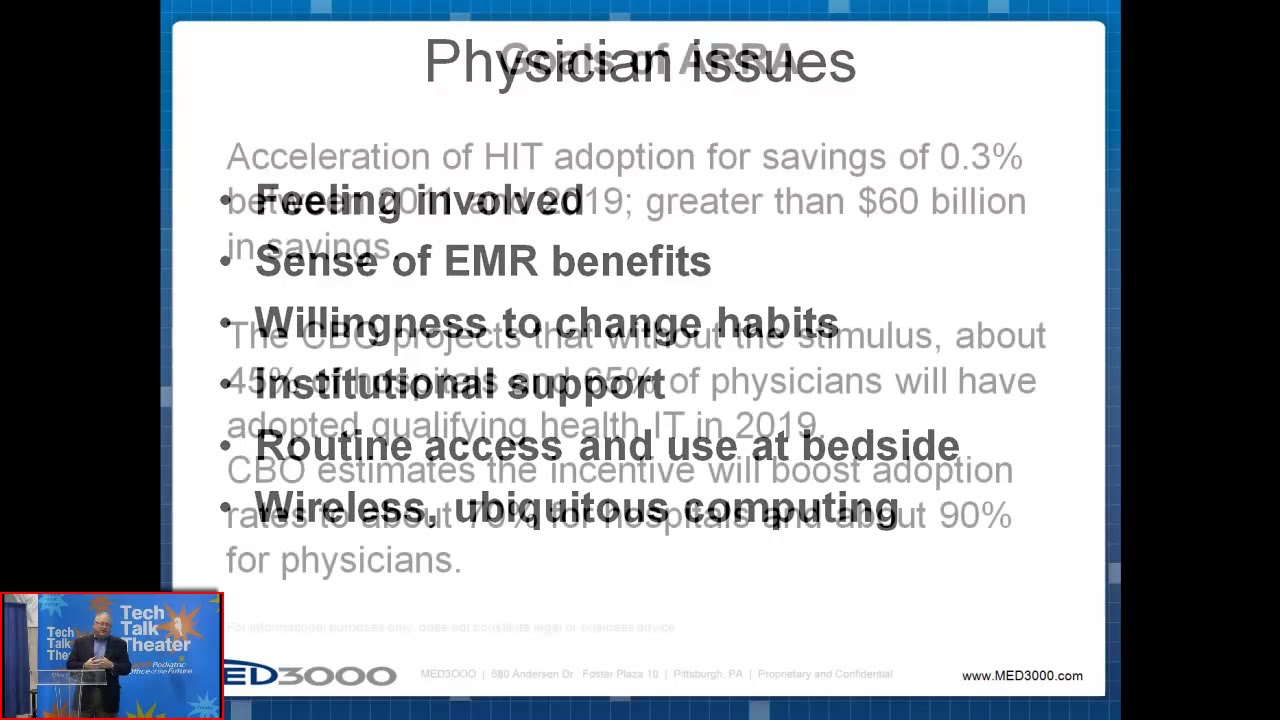The image depicts a PowerPoint presentation slide where two slides are mistakenly superimposed. The prominent text reads "Physician's Issues," with several layers of overlapping text making other parts hard to decipher. Key phrases include "Acceleration of HIT Adoption for Savings of 0.3%," "Feeling Involved," "Sense of EMR Benefits," and hints towards financial impact, such as "greater than $60 billion." Additional text mentions "willingness to change habits," "stimulus about physicians adopting qualifying health IT in 2019," "institutional support," "routine access and use at bedside," "CBO estimates the incentive will boost adoption," and "wireless ubiquitous computing." In the bottom right of the image, there's a smaller photo of an elderly man in a suit and bow tie giving a speech at a clear dais, with "Tech Talk Theater" written in the background. This setup suggests a multimedia presentation possibly being displayed at a tech conference or similar event.